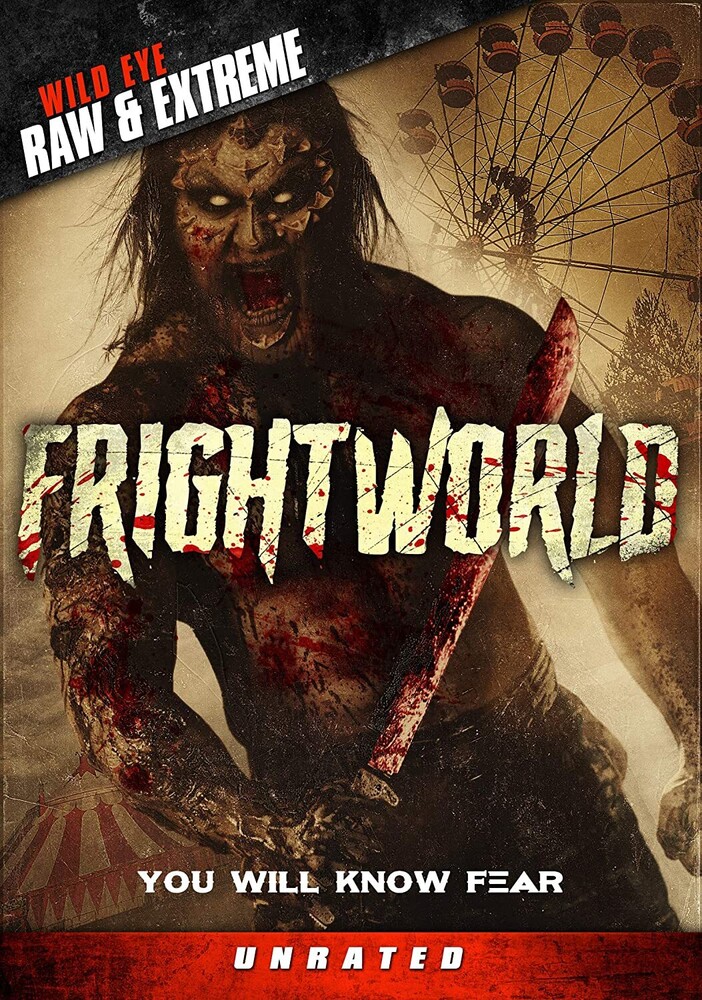The image is a graphic promotional movie poster with an overall dark, gloomy, and spooky theme. Dominating the center is large tan-colored text reading "FrightWorld" as one word. Behind this text looms a terrifying zombie-like creature covered in blood. This creature, shirtless and wearing dark pants, wields a bloody machete in his right hand. He has straggly long hair, white eyes outlined in black, and an open, blood-filled mouth as if screaming. Blood splatters partially obscure the text. 

In the background, to the upper right, a ferris wheel is visible, hinting at a carnival or theme park setting. Additional subtle details include a merry-go-round in the lower left and a carnival tent, reinforcing the eerie amusement park atmosphere. 

Text elements in the poster include a red banner at the bottom stating "Unrated," likely indicating the movie's rating status, with the tagline "You Will Know Fear" just above it. In the top left corner, additional text reads "Wild Eye, Raw and Extreme." The predominant colors across this chilling scene are shades of tan, red, white, black, and gray.